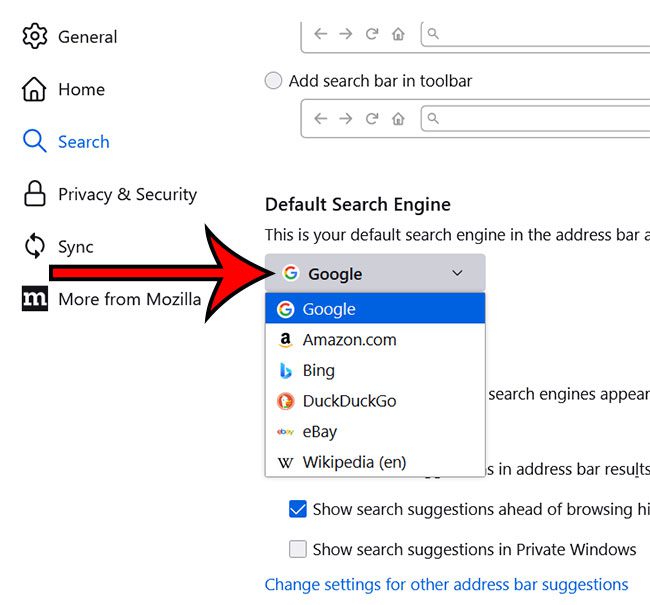**Detailed Caption:**

This is a screenshot showcasing the settings menu of an application or website, featuring a clean white background. On the left side of the image is a vertical list of options, each accompanied by an icon:

1. At the top, there is a gear icon labeled "General".
2. Below it, a house icon with the label "Home".
3. Next, an icon of a magnifying glass with the label "Search," which is highlighted in blue, indicating it is currently selected.
4. Following that is a lock icon with the label "Privacy and Security".
5. Underneath is a refresh symbol consisting of two arrows in a circle, labeled "Sync".
6. Lastly, near the bottom, a black box with a white "M" inside and the text "More from Mozilla".

On the right side of the image, above this menu, a red arrow points to a drop-down menu beside the text "Default Search Engine". The accompanying text explains, "This is your default search engine in the address bar."

In the drop-down menu below, the search engine options are listed in this order:
- At the top, in gray text, is "Google".
- Below that are other options including "amazon.com," "Bing," "DuckDuckGo," "eBay," and "Wikipedia".